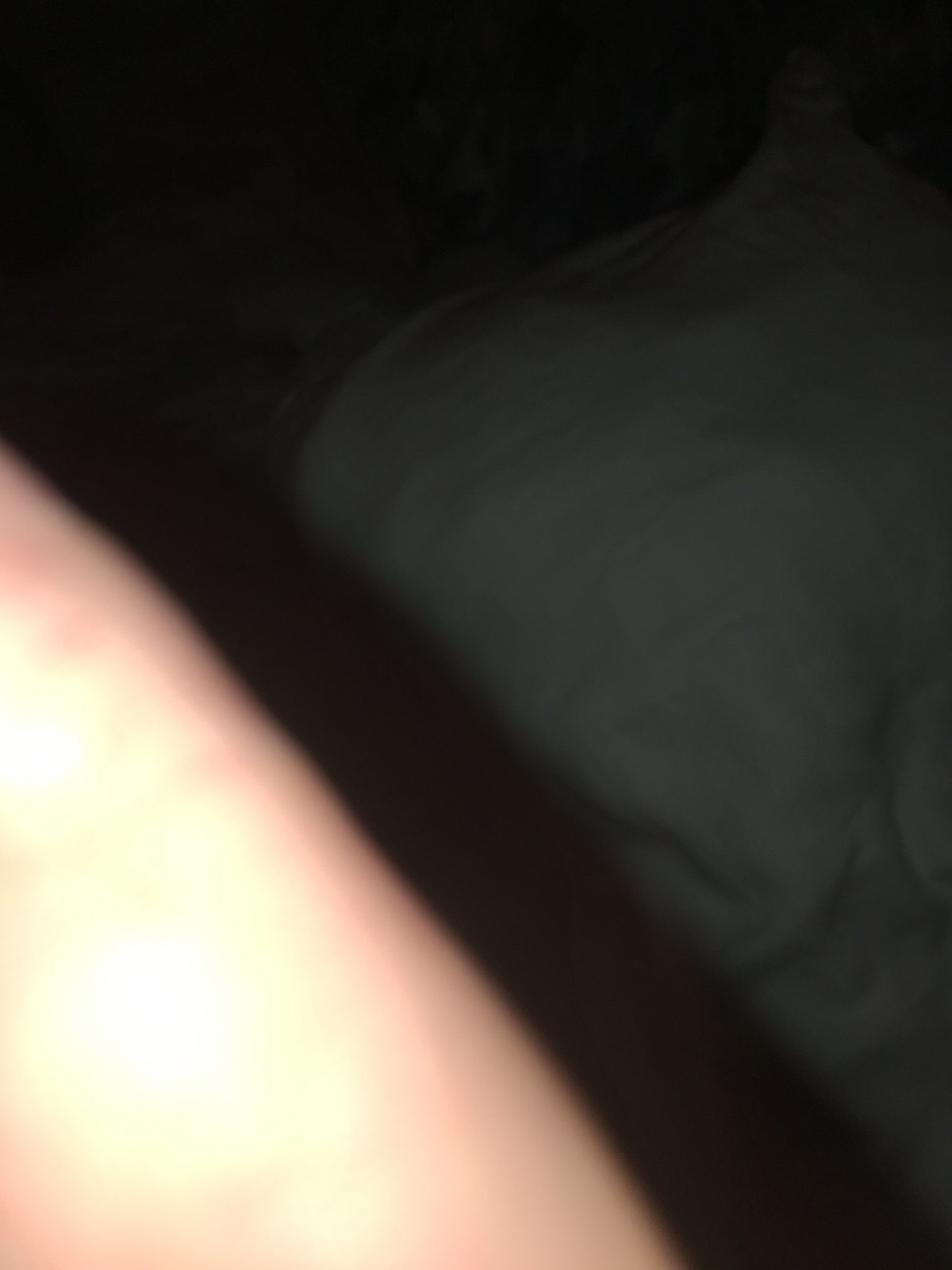The image is notably obscured and blurry, presenting a challenging scene to decipher. On the right-hand side, there appears to be a white object resembling a pillow, possibly resting on a bed. The bed could be framed by wood, or alternatively, it might be a wooden table adjacent to the pillow. On the left-hand side of the image, a pinkish-peach hue is visible, likely representing a blurred arm. The edges of this arm are extremely out of focus, adding to the overall indistinctness of the photograph.